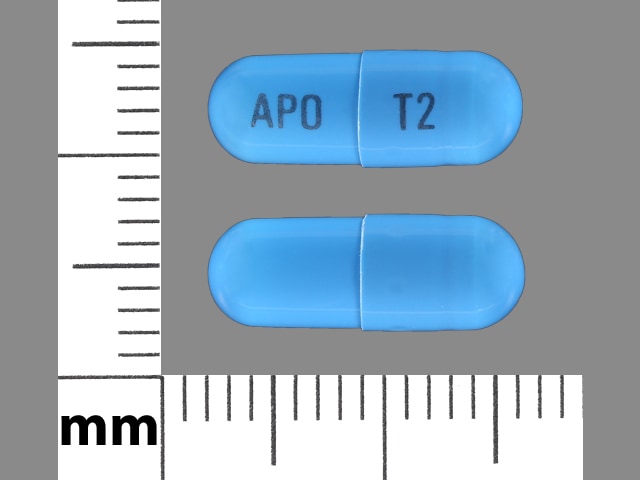The image displays a section of a webpage with information about medication, set against a grey background. The foreground features a millimeter ruler forming an L-shape, extending from top to bottom and then horizontally from left to right. The ruler, marked only with millimeter measurements and delineated by long and short lines, has the "millimeters" label located in the bottom left corner.

Centrally, the image showcases the front and back view of a blue pill capsule. The capsule is vibrant in color, with its halves clearly demarcated. The top half of the capsule is imprinted with the text "APO" on one side and "T2" on the other side. The capsule dimensions are detailed: approximately 2 millimeters long, 2.5 millimeters wide, and slightly more than 0.5 millimeters in diameter.